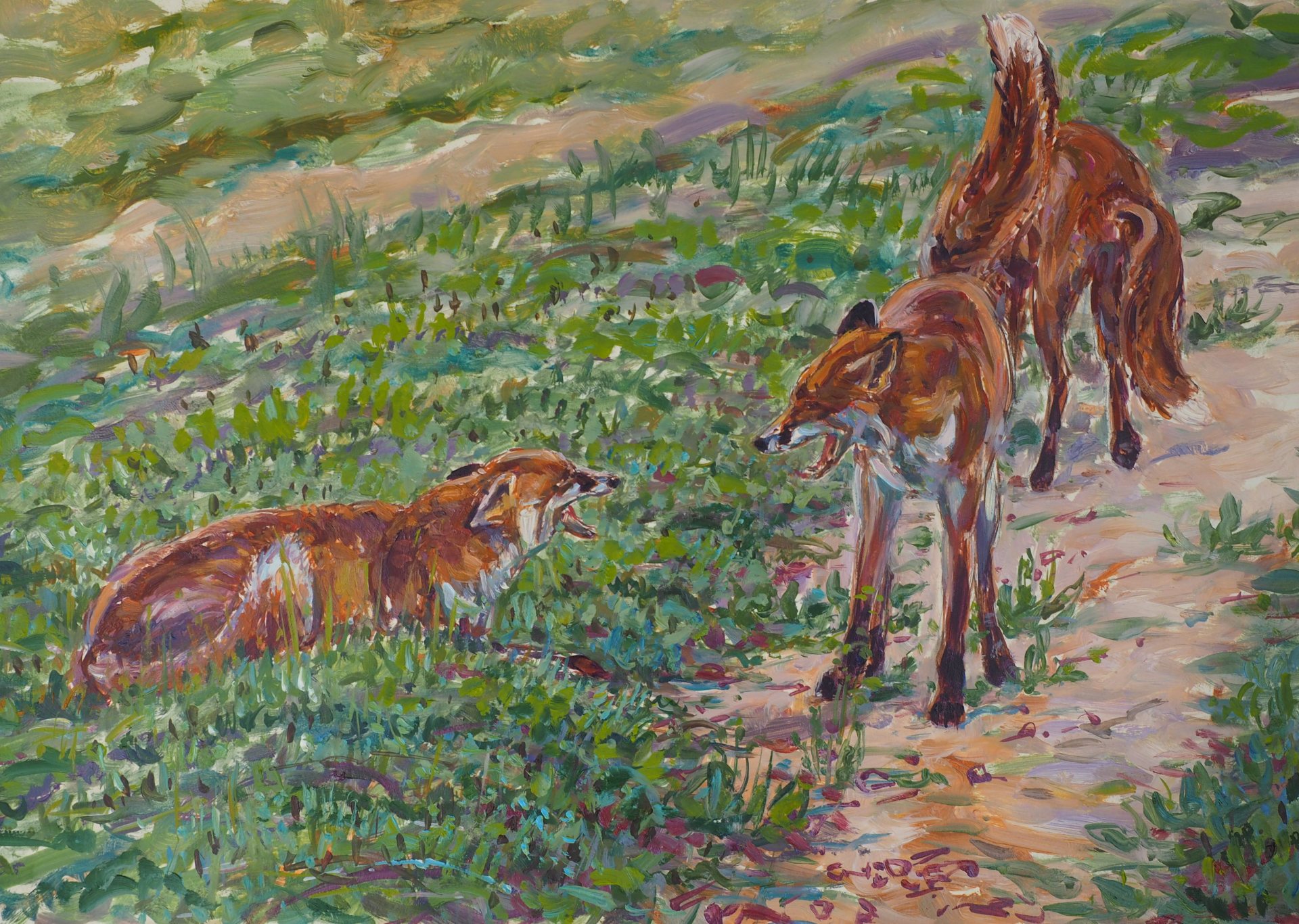The painting is an impressionist-style depiction of three red foxes with white faces, underbellies, and tail tips, set in a contrasting environment of dirt and grass, accented with hints of purple and red flowers. The central focus is on a tense interaction among the foxes. The fox on the left side of the frame is laying in a patch of grass, growling with its ears lowered, while facing two standing foxes to the right. One of the standing foxes, positioned slightly forward on a dirt pathway, appears more aggressive with its mouth open, displaying its sharp jaw. The third fox, situated behind the aggressive one, has its back turned to the viewer, partially obscured by the other fox's upright tail. The hurried and rushed brushstrokes and the blend of colors add to the dynamic and somewhat fierce atmosphere of the scene, despite the otherwise peaceful nature of the landscape.